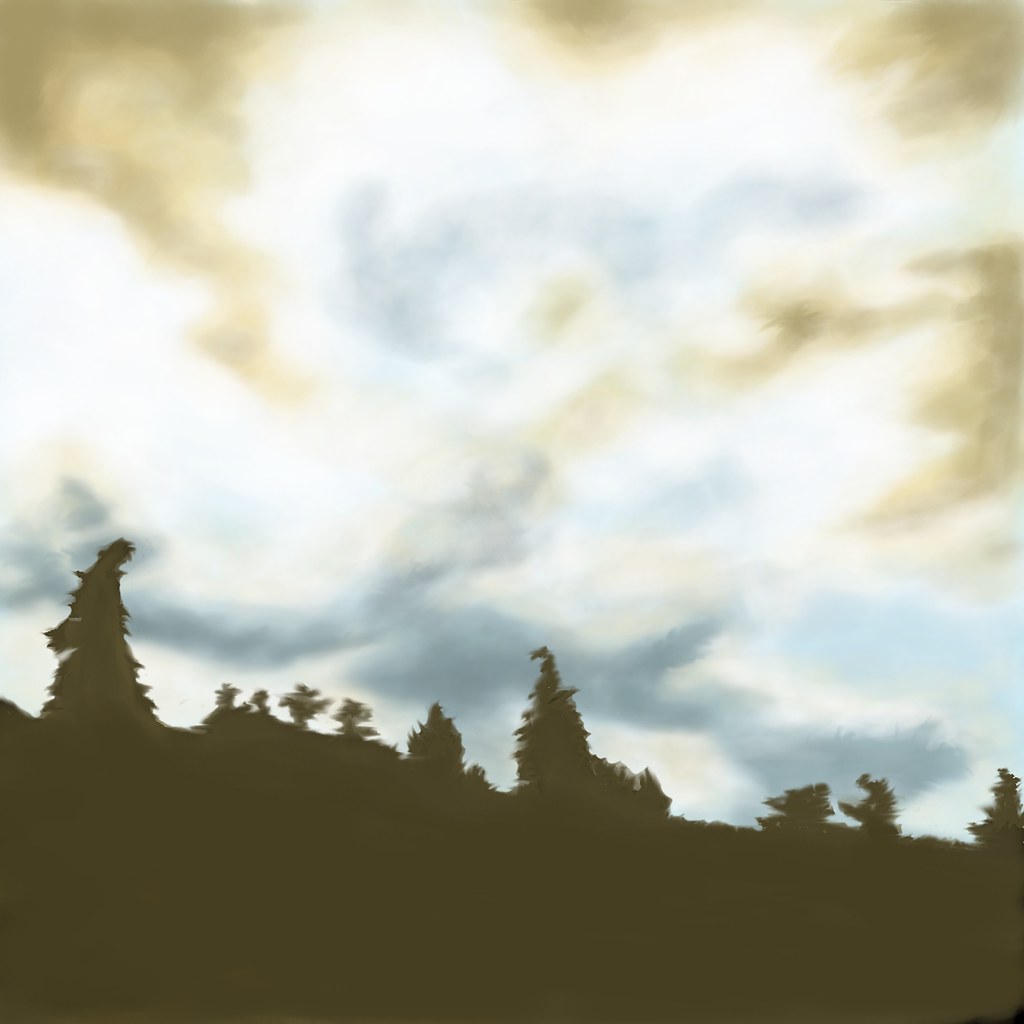This digital artwork presents a captivating view from a low vantage point, gazing up towards the crest of a hill. The land and trees form a striking silhouette, rendered in a solid, earthy brown. Above the hill, the sky is alive with dynamic clouds, depicted in varying shades of white, blue, yellow, and beige. The watercolor effect of the clouds adds depth and texture, with the colors transitioning from a cooler grey-blue at the base to warmer yellows near the top and edges. The overall composition creates a sense of serene beauty and elevation, capturing the blend of natural elements and artistic expression.